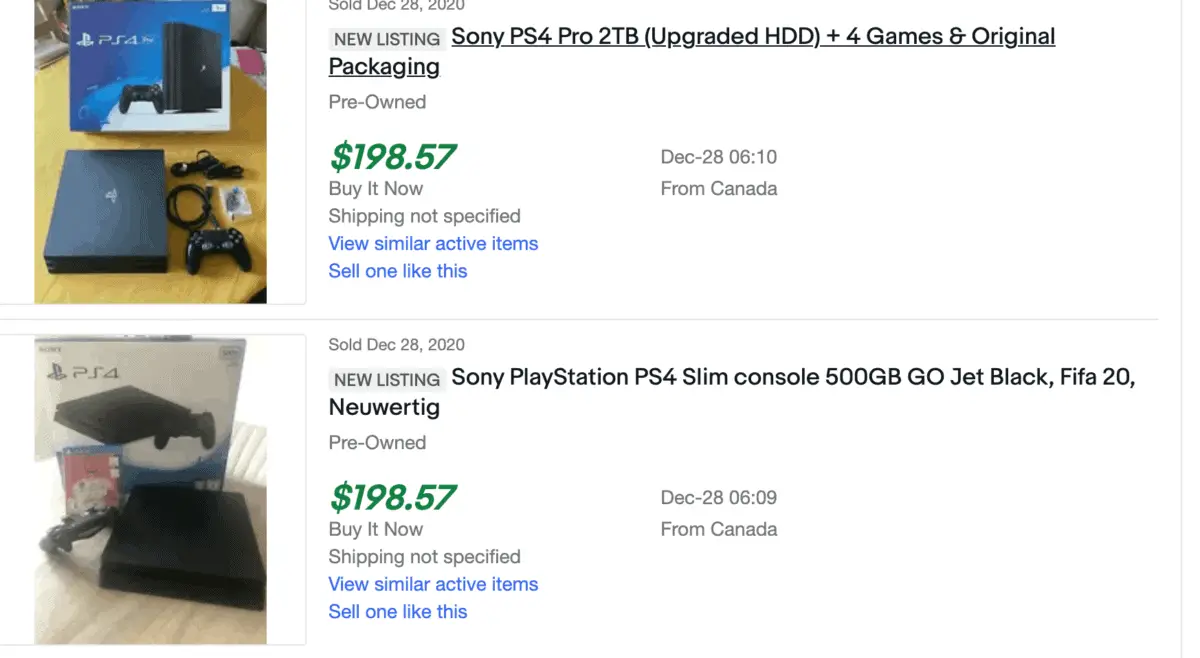The image displays a webpage featuring listings of video game hardware for sale, specifically focusing on Sony PlayStation consoles. On the left-hand side of each listing, there's an image corresponding to the product being sold.

1. The first listing showcases a Sony PlayStation 4 Pro with 2 terabytes of upgraded HD storage, including 4 games and the original packaging. The image depicts the console's box, along with the included games and controllers. This item is marked as pre-owned and was sold on December 28, 2020, for $198.57. Below this listing, there are blue links labeled "View similar active items" and "Sell one like this."

2. The second listing features a Sony PlayStation 4 Slim console with 500 gigabytes of storage, in Geo Jet Black, bundled with "Fifa 20" and a game titled "Warteg." This item is also pre-owned and listed at the same price of $198.57. It too was sold on December 28, 2020. The left side image shows the actual PS4 Slim console. Similar to the first listing, it provides blue links at the bottom for "View similar active items" and "Sell one like this."

The webpage's design emphasizes the visual representation of the products and includes key details for potential buyers, such as the condition of the items, price, and sale date.